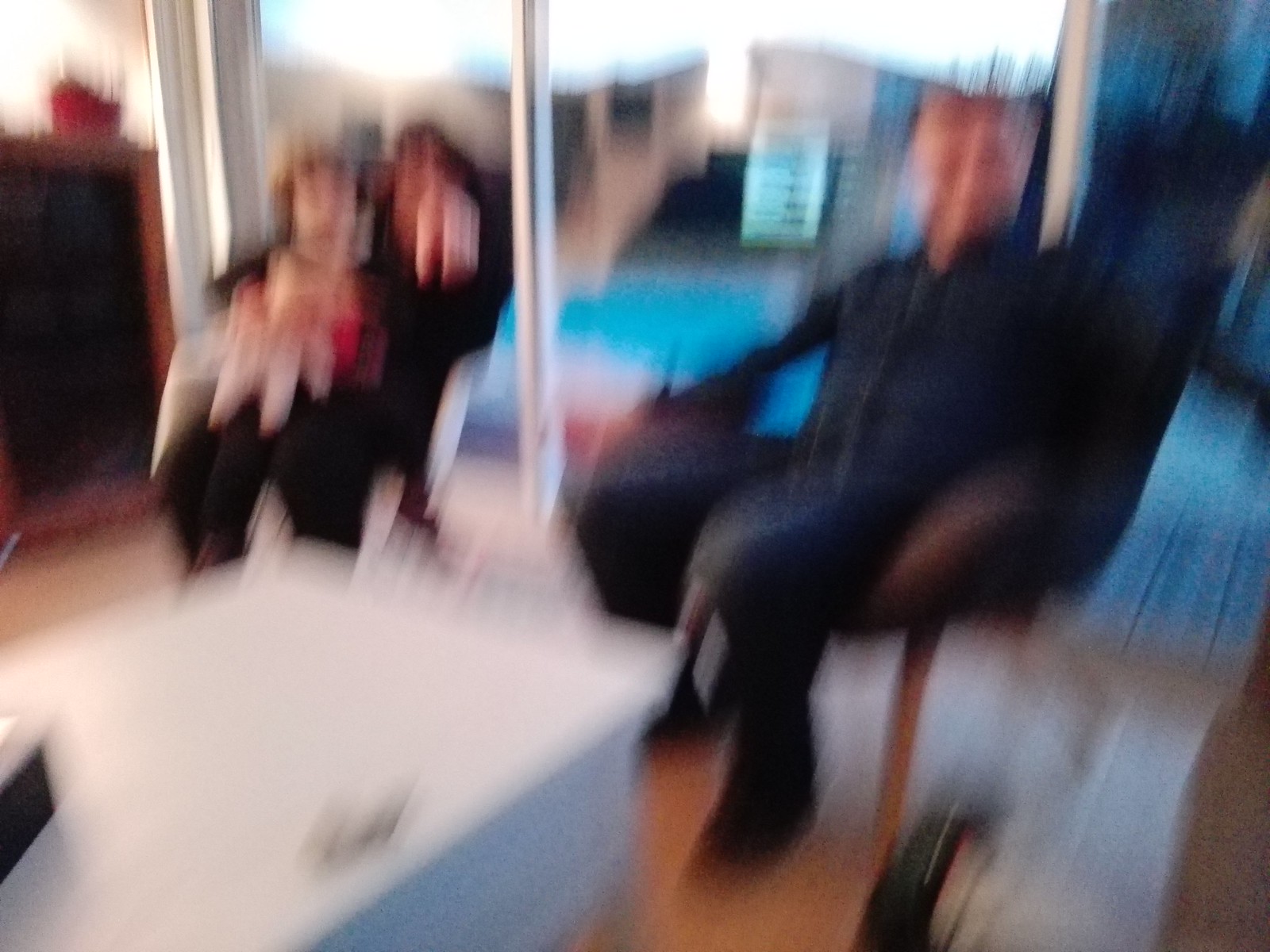In this blurry photograph, a small group of people is sitting indoors on light brown wooden flooring, gathered around a low, white knee-level table. The scene appears to take place in a living room. On the right side, a person in a black chair is dressed in a blue shirt and matching blue pants, attentively looking towards the camera. To the left, another person wearing a black jacket, a red shirt, and black pants sits in a separate chair with a child on their lap. The child is holding a stuffed animal or doll. Behind them, there's a glimpse of another house through a sliding door, possibly featuring a pool. Also visible is a piece of black furniture positioned to the side, adding to the room's setting.